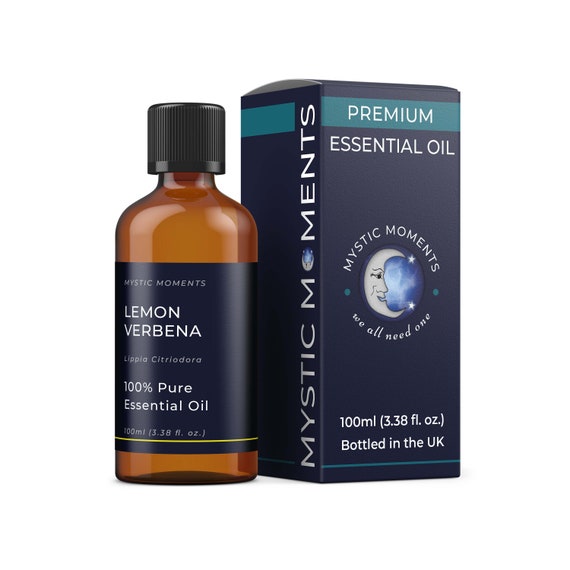The image showcases a meticulously designed product display featuring a bottle of 100% pure Lemon Verbena essential oil and its corresponding case. The brown glass bottle, adorned with a sleek black lid, stands prominently on the left. Its black label, centrally marked with white text, displays the brand name "Mystic Moments" along with "Lemon Verbena, 100% Pure Essential Oil," providing a clear and professional presentation.

Adjacent to the bottle, on the right, is a rectangular black case that complements the bottle's elegance. The case features a stylized branding with "Mystic Moments" written at the top, accompanied by a whimsical white crescent moon logo against a night sky backdrop depicted in shades of blue. Additional text on the package includes "Premium Essential Oil" at the top, "100 ml (3.38 fluid ounces)" in the middle, and "Bottled in the UK" at the bottom, all in white. A teal-colored stripe adorns the top of the package, adding a touch of sophistication to the overall design. The setting suggests a high-end product advertisement focused on premium essential oils.